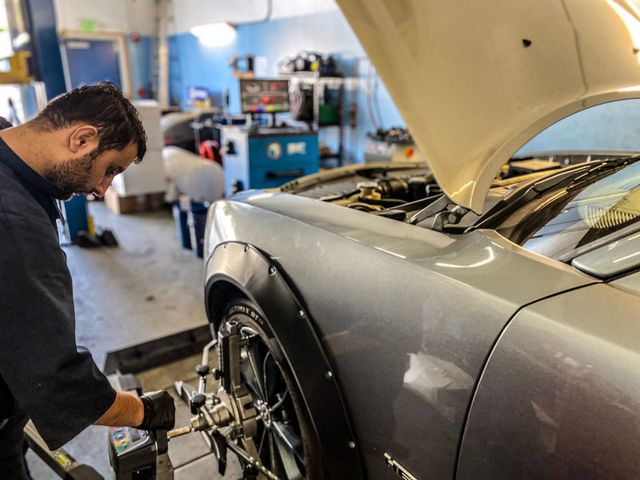The photograph depicts a detailed indoor scene where a car mechanic is diligently working inside a garage. The background is split into a blue lower wall and a white upper wall. Various tools and shelves filled with car parts are visible, accompanied by a blue table with a computer or screen. Partially seen in the upper left corner is a yellow vehicle lift with rods extending upward.

At the center of focus lies a silver car with its hood open, revealing glimpses of the engine. The car, which has black trim around the wheels and appears in good condition, is parked on a reflective cement floor, illuminated by bright lights from above.

A man with short dark hair and a beard, clad in a dark blue uniform and black gloves, is positioned on the left side of the image. He is concentrated on the car’s front wheel, working with a piece of machinery attached to the rim, potentially to secure or remove the tire. The mechanic stands intently, his profile showing as he engages with the tool in his right hand.